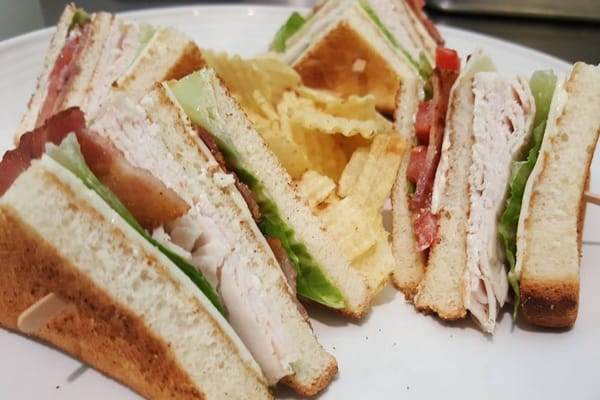This image captures a close-up view of a hearty and vibrant sandwich platter, centered on a large, round white plate. The plate holds four generously-sized quarters of a sandwich, each securely held together by a wooden stick. The sandwiches feature thick slices of toasted white bread, layered with crisp green lettuce, ripe red tomato slices, light-colored deli turkey, bacon, and a slice of cheese, reminiscent of a club or turkey sandwich. Nestled between the sandwich quarters, there's a small pile of wavy, ruffled potato chips. The photograph is focused closely on the sandwiches, filling the frame with their appetizing details and vibrant colors, with only a hint of a metallic background, possibly a refrigerator, slightly visible but not prominent.